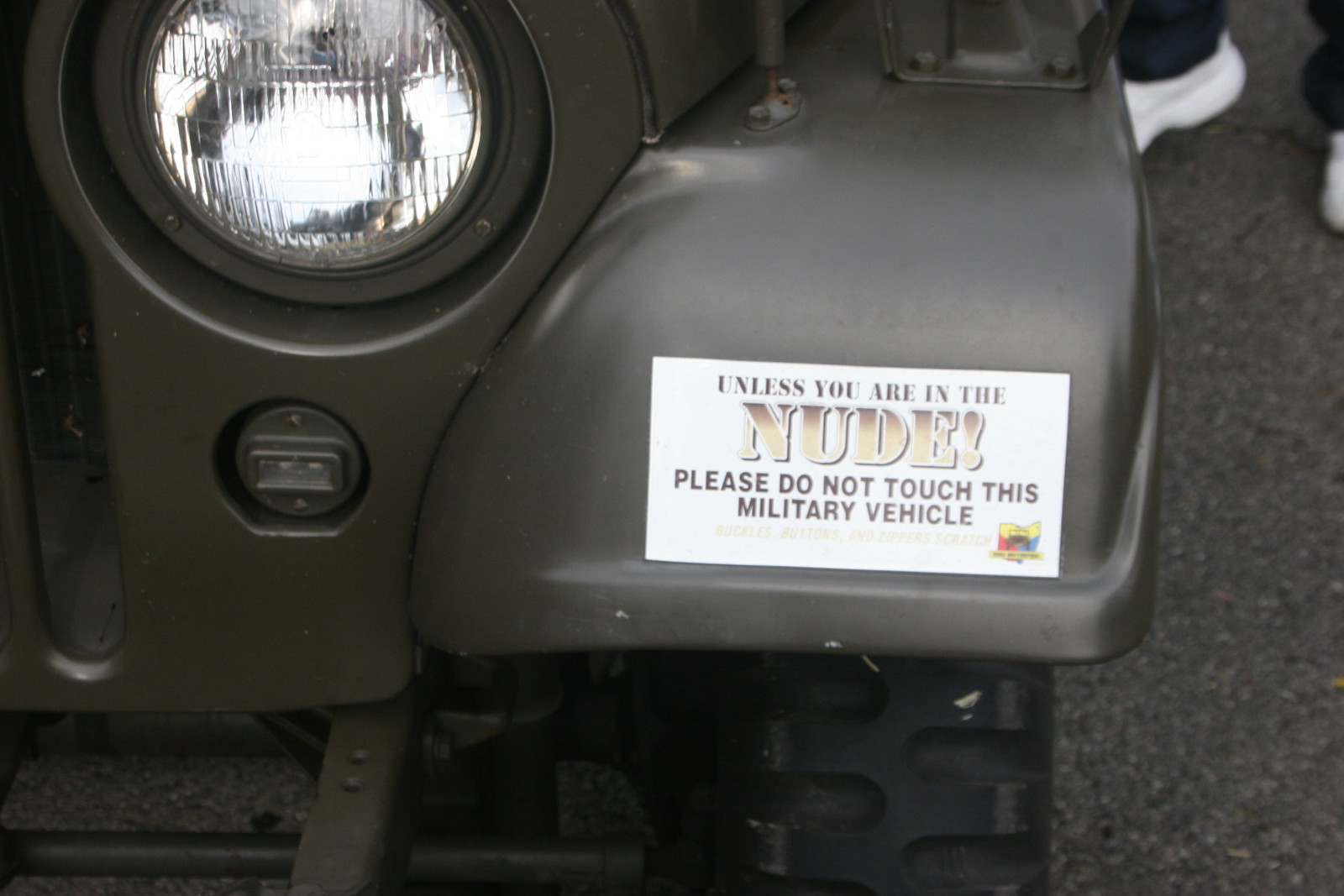The picture showcases a close-up view of the front left wheel guard of a Jeep with classic, rounded details, evoking an old-timey feel. The vehicle is painted in a military green color, suggesting its use or heritage as a military vehicle. Prominently displayed above the small back right tire is a white bumper sticker with a humorous warning: "Unless you are in the nude, please do not touch this military vehicle." The word "NUDE" stands out in large, brown-to-light brown gradient letters, accented with an exclamation point. In the bottom right corner of the sticker, there is a small image of the state of Ohio, hinting at its location or ownership. Also visible in the image are a circular headlight on the vehicle and the white sneakers of an onlooker, adding context to the scene which is set on a paved surface. The backlight of the vehicle, either yellow or white, can be seen but is not illuminated. This Jeep, possibly on display or owned by someone from Ohio, merges historical design with a touch of humor.